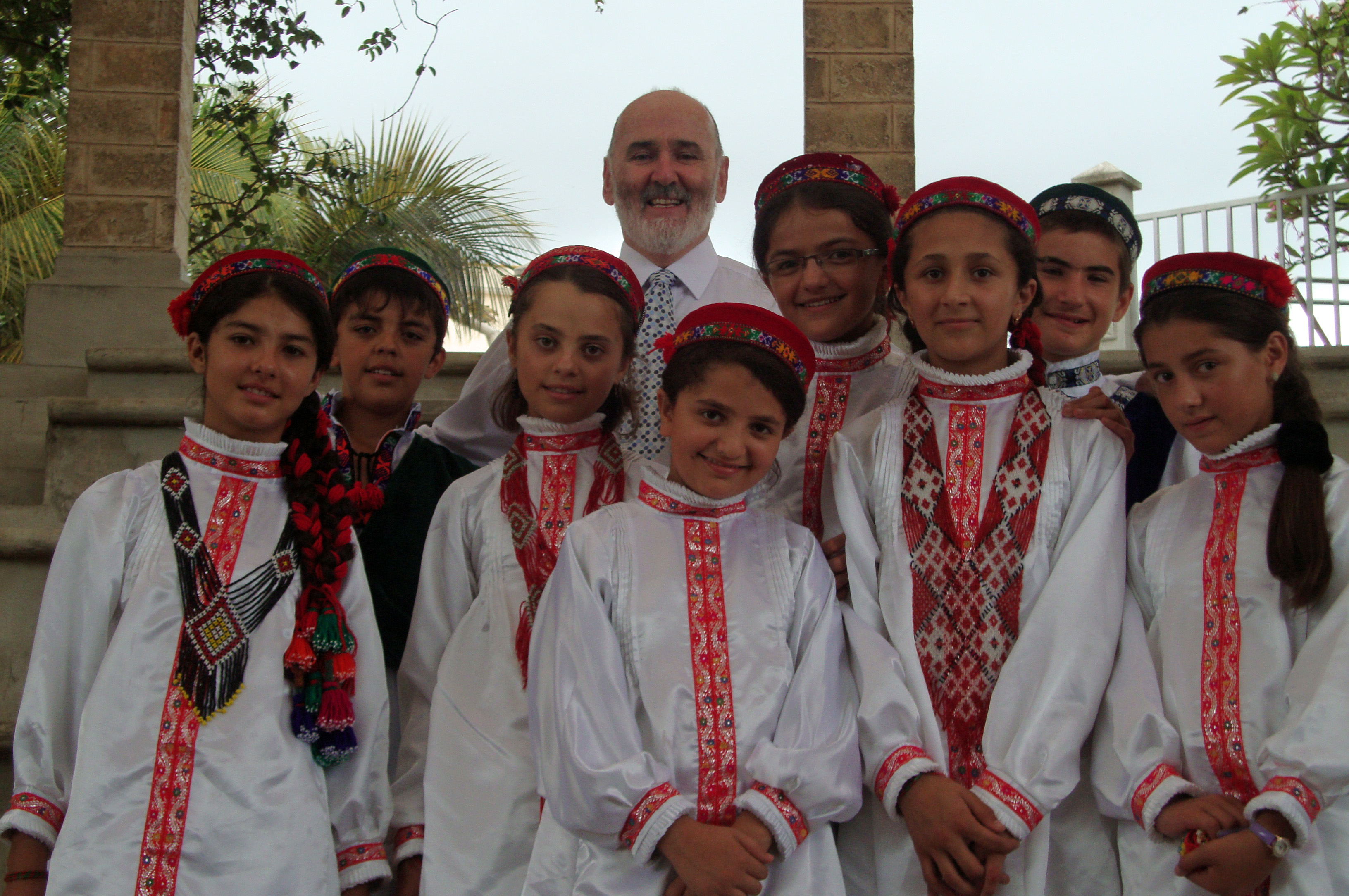In this vibrant and cheerful group photo, a diverse group of eight children, aged around eight to twelve years old, and one older man is captured against the backdrop of a clear blue sky, with trees and bushes adding a natural touch to the scene. The children, comprising six girls and two boys, stand in a neat row, with the shorter ones in the front and the taller ones at the back, ensuring everyone's face is visible and all are smiling at the camera.

The children are adorned in traditional attire featuring long white dresses with puffy sleeves, each embellished with a red strip running down the center adorned with intricate gold geometric patterns. Around their wrists and collars, these dresses have additional red detailing, including floral designs. Some children are also adorned with red scarves featuring checkered designs and circular red headbands with colorful patterns around the base. The girls uniformly sport red headbands, while the boys wear darker hats, possibly black or green.

The man standing behind the children, sporting a bald head, white beard, and gray mustache, is likely their teacher, mentor, or guide. He is dressed in a white button-down shirt paired with a checkered blue, gray, and black tie, adding a formal touch to the gathering.

This well-composed image is set outdoors in front of a stone wall and gate framed by two narrow brick pillars, enhancing the cultural and traditional aesthetic of the scene.